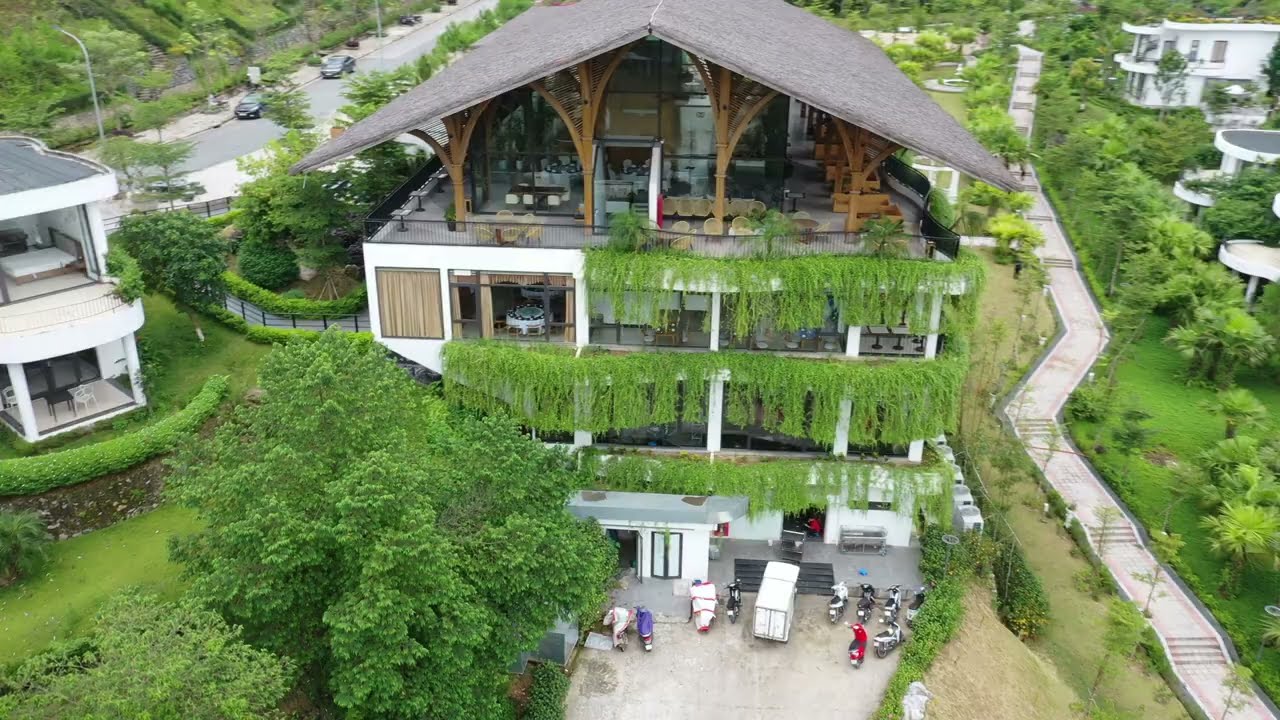The photograph depicts a grand, multi-story building, possibly a residence or hotel, reminiscent of an Asian-inspired design. The structure, approximately four to five stories tall, is adorned with lush green vines draping from the first three floors. The flat rooftop supports an additional structure with a distinctive black triangle roof held up by brown bamboo wood beams, evoking a tropical or thatched look. The front facade features expansive glass windows and white columns, with a balcony on the top level providing ample seating with light-colored chairs and tables. 

In the yard, there are numerous motorcycles in various colors, a white trailer, and an assortment of other items. The left side of the building is framed by tall trees, bushes, and grass, and a two-story white house is visible nearby. The right side reveals a long stairway or walkway bordered by park-like greenery, leading to more two-story white houses with gray rooftops. Beds, tables, and chairs are visible through the see-through windows, adding to the residential feel.

The backdrop includes a road with streetlights and parked cars, surrounded by additional greenery and benches. The street, lined with trees and bushes, further enhances the scene, highlighting the upper-class ambiance of this residential area.